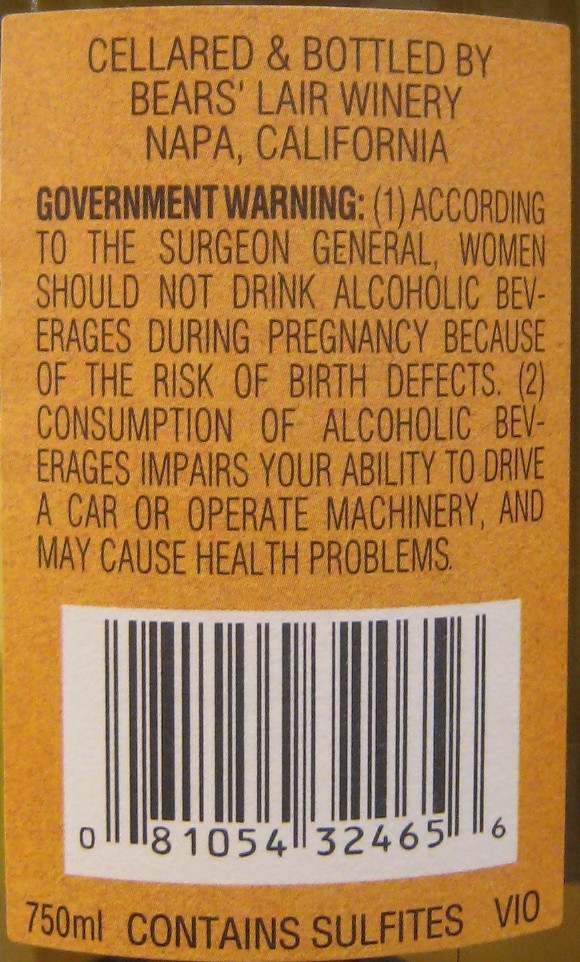The image shows an older wine bottle label with a rustic and faded orangish-yellow background. At the top, it reads "CELLARED AND BOTTLED BY BEARS' LAIR WINERY," followed by "NAPA, CALIFORNIA," all in capital letters. Below that, in bold, it presents a government warning: "(1) According to the Surgeon General, women should not drink alcoholic beverages during pregnancy because of the risk of birth defects. (2) Consumption of alcoholic beverages impairs your ability to drive a car or operate machinery and may cause health problems." Beneath this warning, there is a traditional barcode with the number "081054324656." At the bottom left, it states "750 MILLILITERS" and "CONTAINS SULFITES" in big capital letters. Towards the bottom right, it is marked with "VIO."